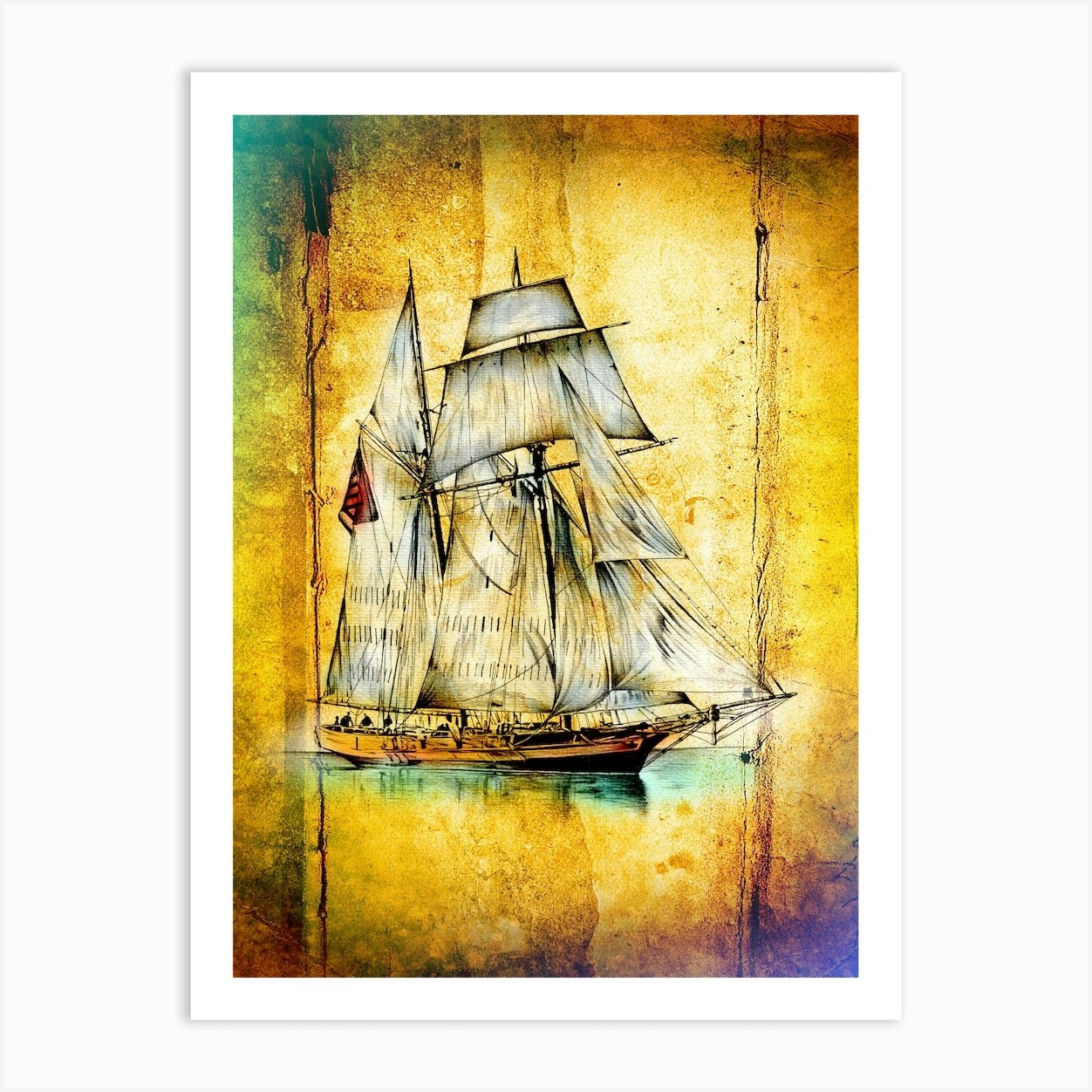This image is a detailed illustration of an old sailing ship, reminiscent of a schooner from the 1700s or 1800s. The ship, adorned with multiple white sails, has a brown wooden body with black stripes. An American flag is prominently displayed, further emphasizing its historical design. While the illustration itself is contemporary, it has been intentionally textured to mimic an aged, weathered appearance, complete with yellowish stains and hints of blue coloring. The ship is set against a yellow background with purple and green corners, adding vibrant accents. The entire piece is bordered by white and gray, framing the image nicely in a nautical, naval theme. A shadow of the ship adds depth to the composition, enhancing its visual appeal.